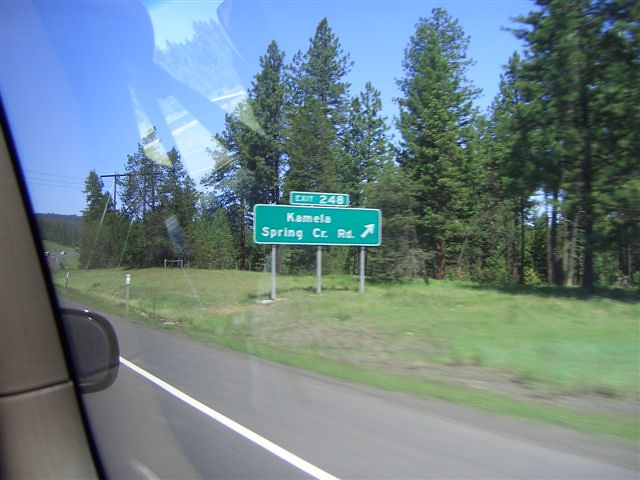A photograph captured from inside a moving car as it travels along a highway. The image prominently features a green highway sign indicating Exit 248 for Camilla Spring Circle Road, with an arrow directing traffic to the right. In the background, a lush stand of evergreens stretches across a rolling grassy hill, framing the scene with natural beauty. Overhead, power lines traverse the sky, casting a geometrical pattern over the blacktop freeway below. The photographer includes a subtle reflection of the car's interior on the window through which the shot was taken, offering a glimpse of the passengers inside.